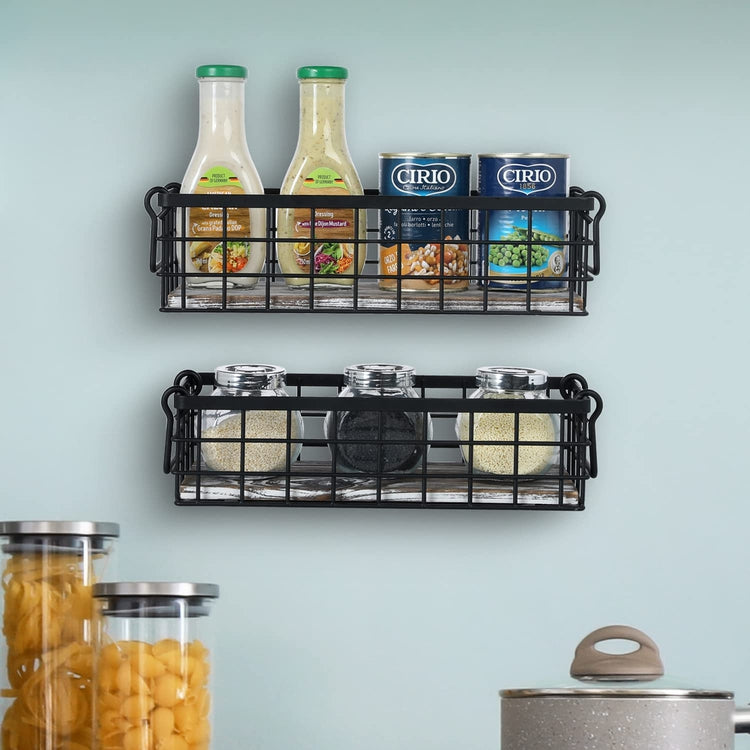The image depicts a kitchen with a light blue wall, featuring two black, metal bar shelves with small handles on either side. The overhanging shelves have three rows of bars for support. The top shelf displays two jars of salad dressing, one filled with a lighter-colored substance, possibly ranch, and the other with a darker yellow dressing. Alongside these jars are two containers of beans, one darker and one green. Below, the bottom shelf holds three round glass spice jars with silver tops; the leftmost jar contains a white spice, the middle jar a black spice, and the rightmost jar another white spice. Underneath this shelf, two clear, vacuum-sealed glass containers are visible, one filled with long pasta like spaghetti or fettuccine, and the other with shell pasta. In the bottom right corner of the image, there is a pot with a brown glass lid, adorned with brown and white speckles. The kitchen is illuminated by light coming from the right side of the image.